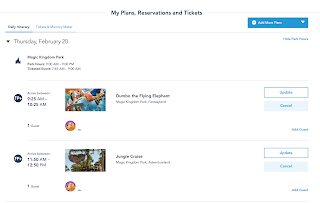This is a detailed screenshot of a website featuring a predominantly white header. There is a thin, white-gray line running horizontally across the entire width of the page, except for a break in the center occupied by some black text. The text begins with the word "My," followed by a blurred second word, and then reads "Reservations and Tickets" to the right. Below and to the right of this text is a noticeable bright blue button. This button displays a white circular icon on the left and some unreadable white text next to it, with a white downward-pointing triangle on the far right end of the button.

Beneath and to the left of this section, there are two underlined words in black text, although they are also unreadable due to blurriness. To the right of these words, there are four additional words in blue text that are similarly blurred and unreadable. Directly underneath this text is a medium-width, light-gray outline, accentuated by another horizontal thin light-gray line extending to the right and almost covering the full width of the page.

Further down, towards the right, there is a line of blue text that remains blurry and unreadable. Adjacent to the left side of this section, there is a black downward-pointing triangle, followed by black text that reads "Thursday, February 20." Below this, the page is partitioned into three distinct sections on a white background, each separated by thin, light-gray lines indented slightly from the left side and extending fully to the right side of the page. Each section includes an icon on the left-hand side, accompanied by corresponding information on the right.